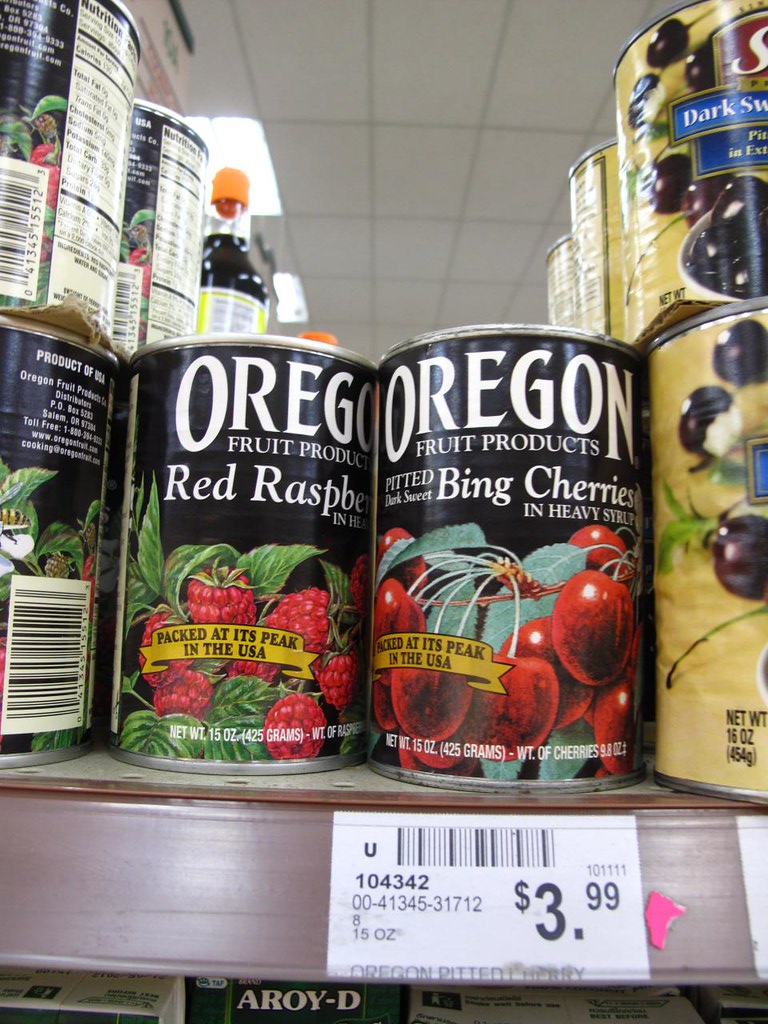A white-tiled ceiling with bright lights illuminates a shelf stocked with various canned goods. The top shelf showcases prominently two black cans with white text that reads "Oregon Fruit Products." The left can features "Red Raspberries" in a vividly illustrated design with raspberries and leaves, while the right can displays "Pitted Dark Sweet Cherries in Heavy Syrup" with corresponding cherry illustrations and leaves. Both cans are marked "Packed at its peak in the USA." Below these cans is a pricing label indicating $3.99 for orange pitted cherries.

Adjacent to these central cans are more products. On the left, a bottle with an orange lid containing a dark liquid stands out. To the right, a set of yellow cans appears to hold other varieties of cherries, possibly dark cherries. Beneath this shelf, another row is visible with a label reading "AROY-D" on a box. The scene provides a detailed glimpse into the well-organized and brightly lit display of fruit products at a retail establishment.